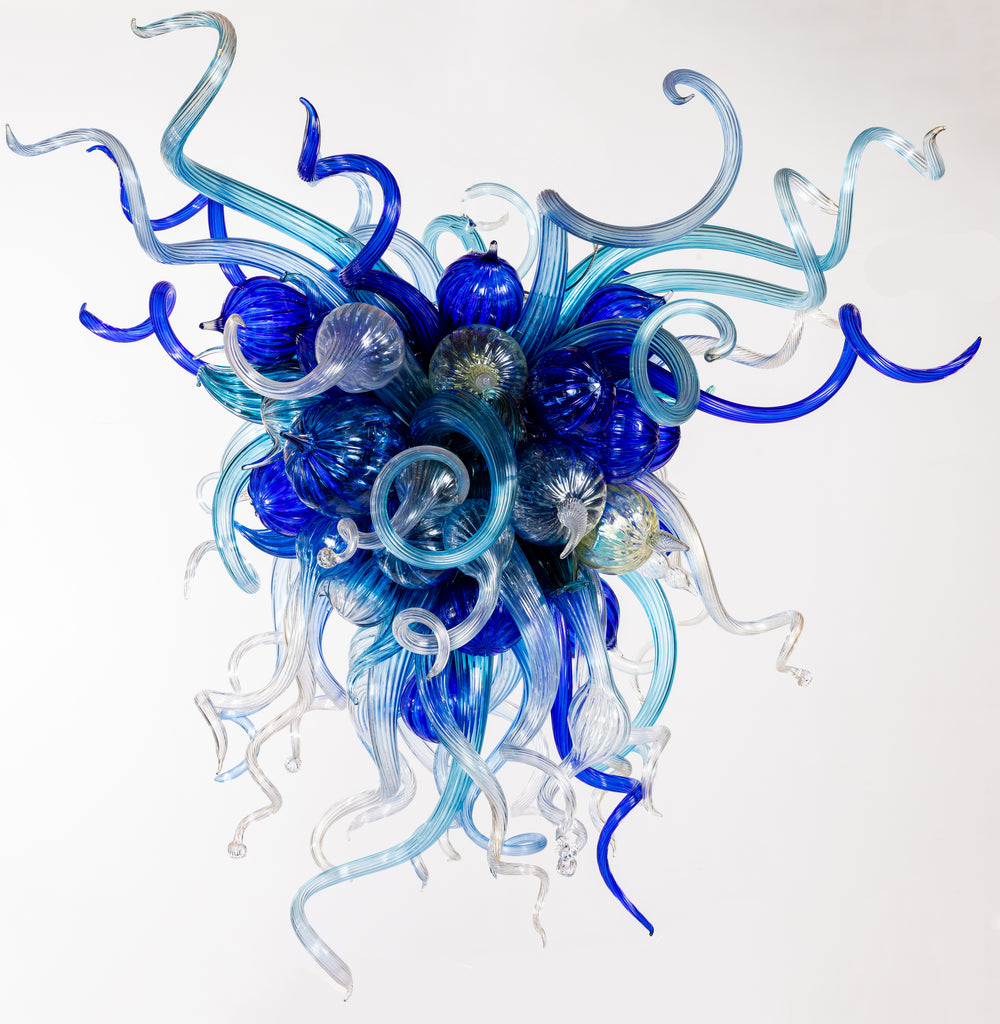The image showcases a hand-blown glass chandelier in the distinctive Chihuly style, featuring a dynamic fusion of shapes and colors against a pristine white background. The modern, abstract glass artwork primarily consists of spirals and twisted protrusions that mimic sea creature tentacles, creating an animalistic appearance. The rich cobalt blue forms the central core of the sculpture, surrounded by lighter shades of baby blue, turquoise, and clear glass. As the sculpture extends outward, the glass pieces become more spread apart, transitioning to translucent whites and turquoise hues. The core structure comprises tightly clustered circular bulbs, reminiscent of a bunch of grapes, with some ending in small knobs and others extending into long, twisting tentacles. This intricate design by Dale Chihuly, dated around 1998, captures the essence of modern glass art and lighting fixture aesthetics in a square format color photograph.